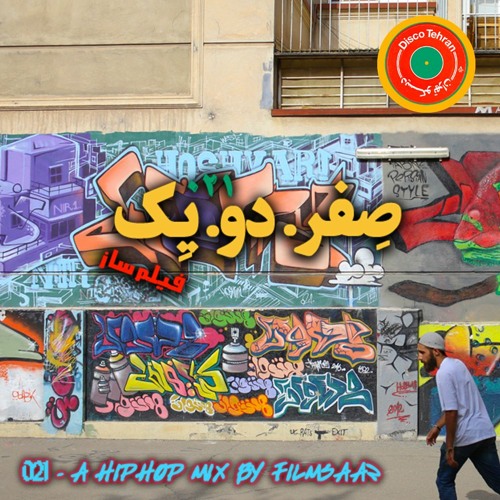This image captures an urban street scene featuring a building adorned with vibrant and diverse graffiti. The photograph, taken from the street, shows the side of a beige-colored building with various layers of street murals. At the top of the image, a balcony with bars is visible, adding a touch of architectural detail to the urban landscape. 

The graffiti spans the entire side of the building, with numerous vivid colors including yellow, red, green, blue, orange, pink, and gray. On the left side of the building, a prominent piece depicts a purple building, overlaid with newer graffiti markings and intricate details. In the center, Arabic letters are painted, adding an exotic and multicultural layer to the artwork. To the right, there is a striking red mask, which stands out among the diverse elements of street art.

Additional pieces of graffiti, characterized by their colorful nature and varied styles, can be seen along the facade and ground level. The lower section of the image captures the sidewalk, where a man is seen leaning forward, presumably skateboarding, although the skateboard itself is not visible in the frame.

At the bottom left corner of the image, text reads, "021, a hip-hop mix by Film Bar," while the top showcases the title "Disco T-Rod." This likely indicates that the image serves as a cover for a YouTube video or a related media project, blending the themes of street art and hip-hop culture.